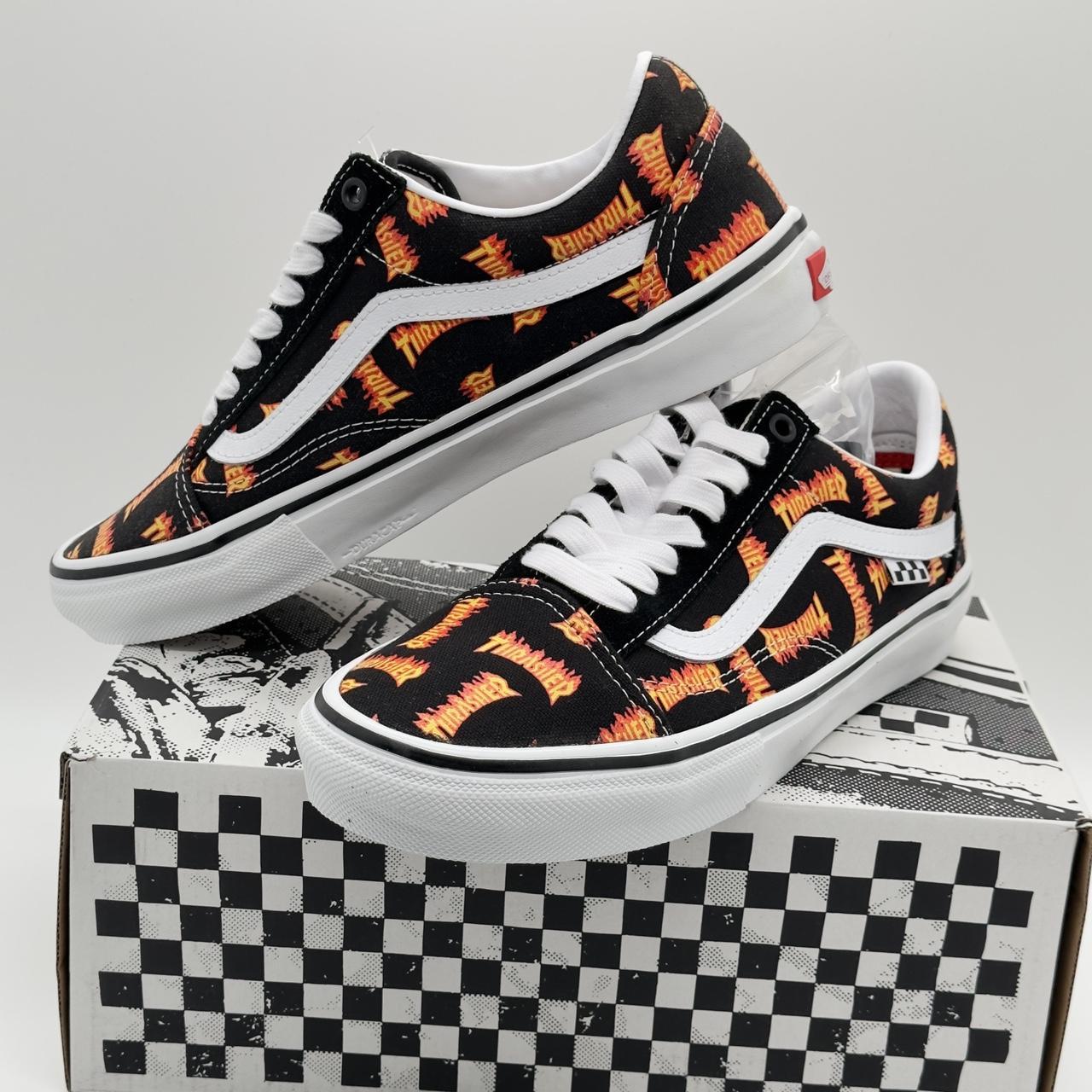The image features a pair of black canvas, low-top Vans tennis shoes adorned with "Thrasher" written in a fiery red and orange script scattered across the shoe. The shoes have signature white laces and white soles with a black stripe running around the base, and also include the iconic Vans white stripe down the side. A partial red and white Vans logo is visible on the back of the shoe. They are displayed on top of a black and white checkerboard-patterned Vans box. The shoes and the presentation suggest a sporty and dynamic aesthetic, typical of a promotional advertisement for a website specializing in selling tennis shoes.